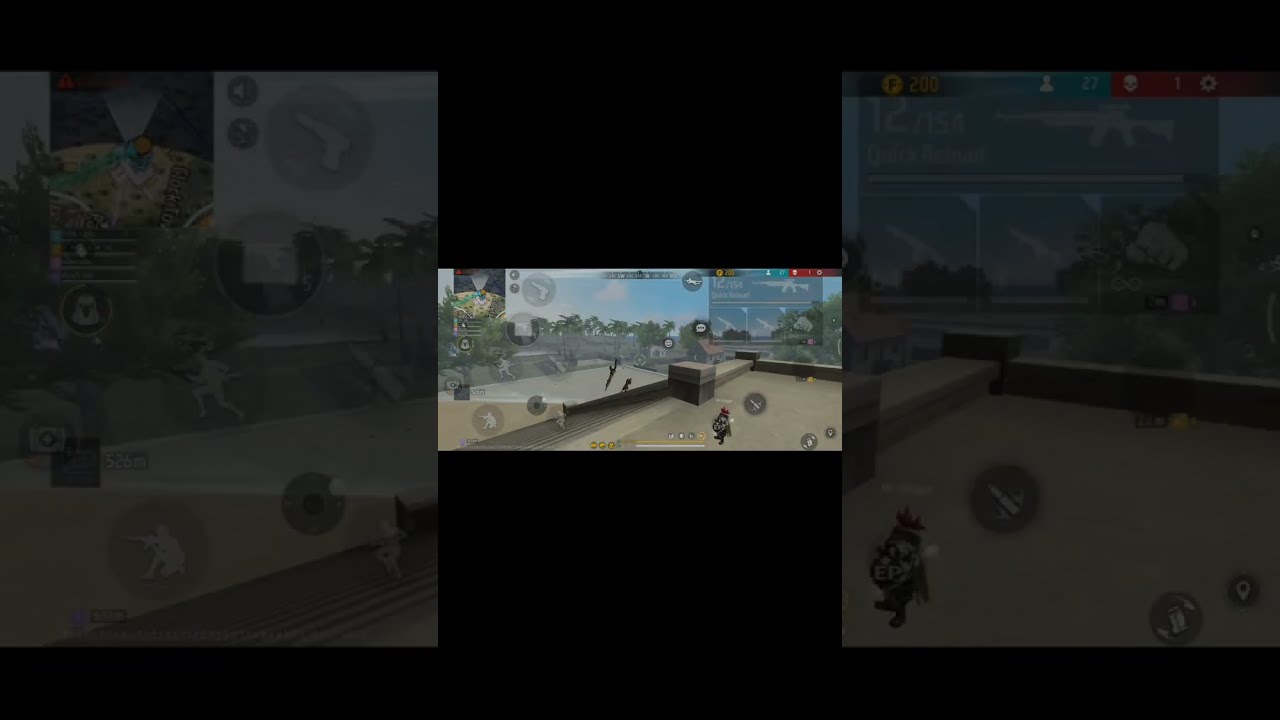The image appears to be a screenshot from a mobile 3D RPG game with shooter elements. In this horizontal screenshot, the main character, adorned in armor with a shield and a sword, is situated on a concrete elevated platform with stairs leading down to a stadium-like area. To the left, there are icons for different movements and actions, such as running, crouching, and switching weapons, indicating a shooter interface. There's an inventory grid and compass visible, enhancing the tactical aspects of the game. The background features a mix of larger and residential buildings, lending a Fortnite-like atmosphere. A distinctive red splotch is noticeable on the top right, possibly a part of the HUD or an alert.